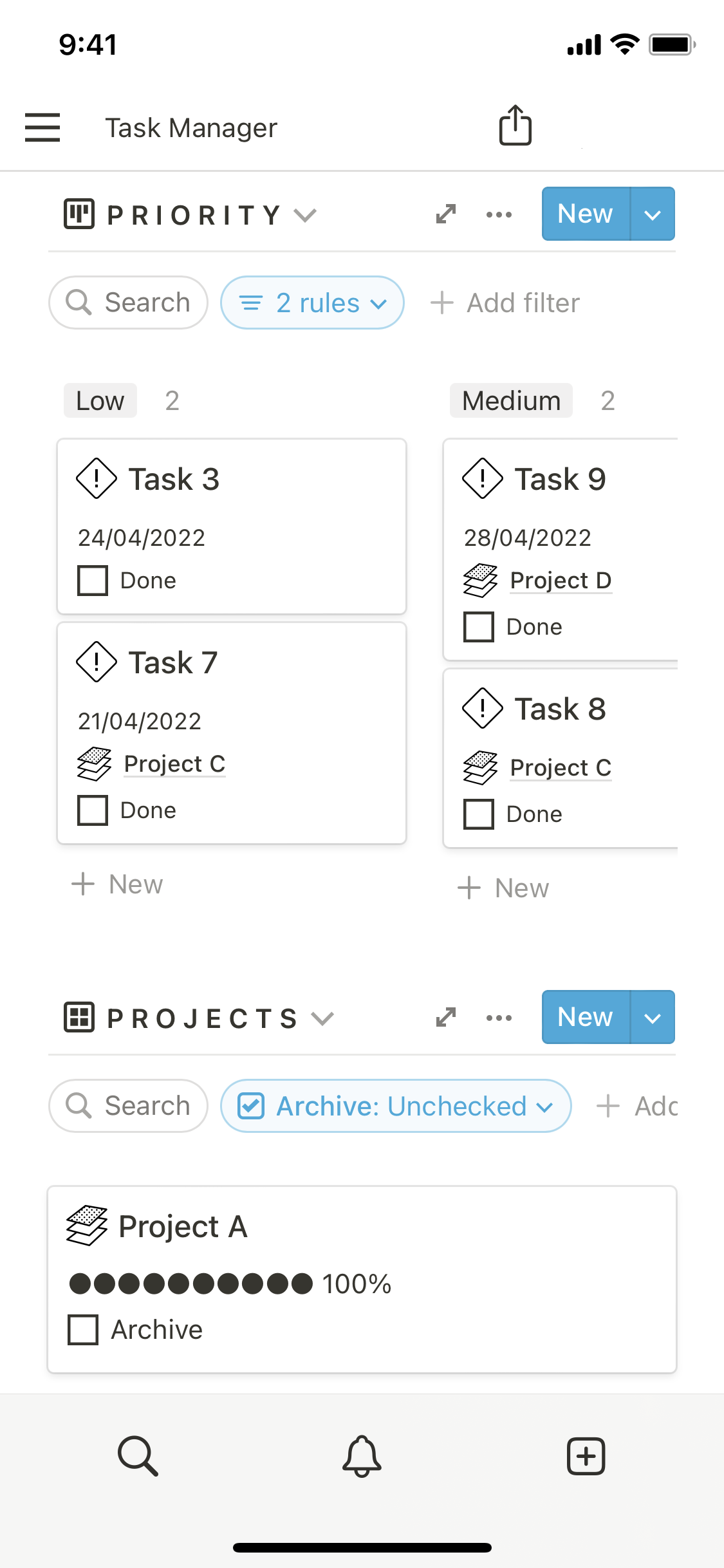This image is a detailed screenshot of a smartphone screen displaying a task manager application interface.

In the top-left corner, the time is displayed as "9:41" without specifying AM or PM. Adjacent to the time, signal strength bars, a Wi-Fi icon, and a partially filled battery icon indicate phone connectivity and battery status.

Under the time display, three stacked bars in black symbolize a menu. Next to this icon, the title "Task Manager" is visible. To the right of the title, there's an icon of a box with an upward-pointing arrow, and beneath this, the text "Priority" appears. Further to the right, there's a dual-ended arrow pointing downward to the left and upward to the right, followed by three vertically aligned dots. Next is a blue box with white text reading "New," accompanied by a downward arrow.

Below these icons is a search bar with a magnifying glass icon and the word "Search" in black. To the right of the search bar, there's a white box outlined in blue with the text "Two Rules" in blue, followed by a plus symbol and the phrase "Add Filter" in black.

Underneath the search area, two gray boxes labeled "Low" and "Medium" with corresponding values "2" are visible. 

The main task display consists of four white boxes, each featuring a black diamond shape enclosing an exclamation point symbol. Each task displays specific details:
- The top-left box reads "Task 3" with the date "24/04/2022" and a "Done" checkbox.
- The top-right box shows "Task 9," the date "28/04/2022," labeled as "Project D," and a "Done" checkbox.
- The bottom-left box indicates "Task 7," the date "21/04/22," labeled as "Project C," and a "Done" checkbox.
- The bottom-right box identifies "Task 8," labeled as "Project C," with a "Done" checkbox.

Below these tasks, a plus symbol followed by "New" appears on both the left and right sides.

The screenshot also includes an additional section with a white box entitled "Project A," listing ten black circles in a row with "100%" next to it. Below this is a black-outlined box labeled "Archive."

Near the bottom, various icons such as a magnifying glass, a bell, and a black outlined box with a plus symbol are present. Finally, a black line runs under the bell icon, demarcating the end of the captured screen.